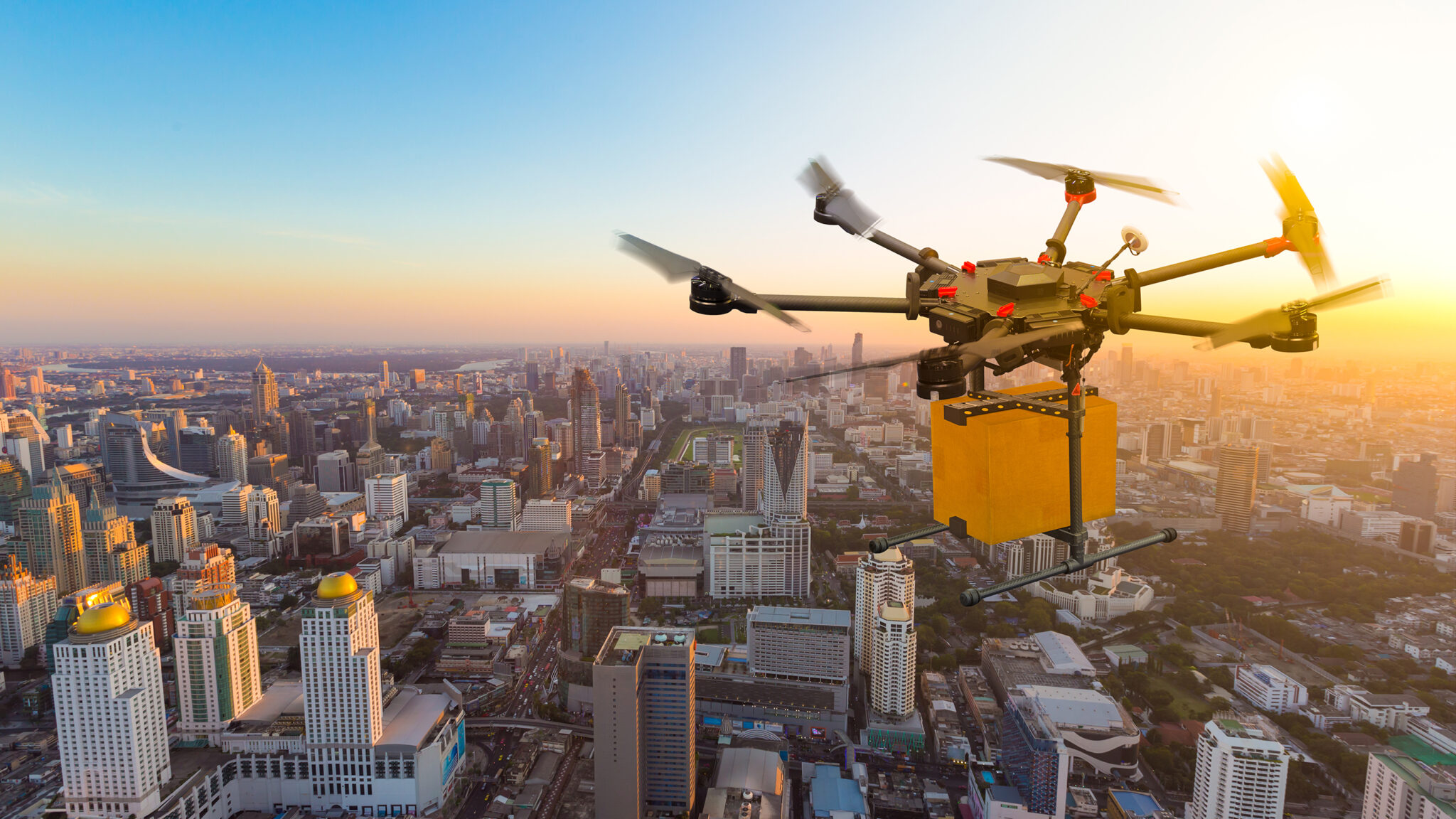The image is a highly detailed CGI rendering of a drone flying above a bustling cityscape. The scene, captured from an aerial perspective, reveals a densely populated urban area characterized by a multitude of tall skyscrapers, roads teeming with cars, flyovers, and even a hint of green space suggesting a park. The city, portrayed as a concrete jungle, emphasizes the convenience of drone deliveries in such crowded settings.

In the upper half of the image, a clear blue and white sky transitions into a picturesque sunset, with the horizon awash in yellow and orange hues, casting a warm glow over the entire scene. The drone, depicted with a hexagonal black body and six propellers, is prominently flying to the right of the frame. Suspended beneath its sleek frame, metal rods hold a yellow-colored package, underscoring the possibilities of rapid, small-item delivery within urban environments. The intricate details of both the drone and the city below highlight a futuristic yet realistic depiction of drone technology in modern logistics.